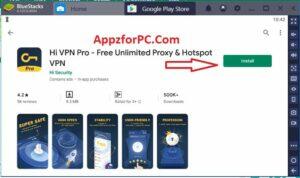In the image set against a white background, there is a small, blurry screenshot with a horizontal orientation. At the top of the screenshot, there are several unreadable tabs. Directly below the tabs is a white rectangle. Centrally displayed on this rectangle is a piece of red bold text: "Apps for PC dot com." Underneath this, in black text, is the phrase: "H-I-V-P-N Pro, Free Unlimited Proxy and Hotspot VPN." To the right of this text is a green action button labeled "Install." On the lower left side of the image, there are five indistinct phone screenshots. These screenshots exhibit a black and gray color scheme with yellow text, but the details are illegible. On the right side of the image, several white icons are set against a black background; however, the specifics of these icons cannot be discerned.